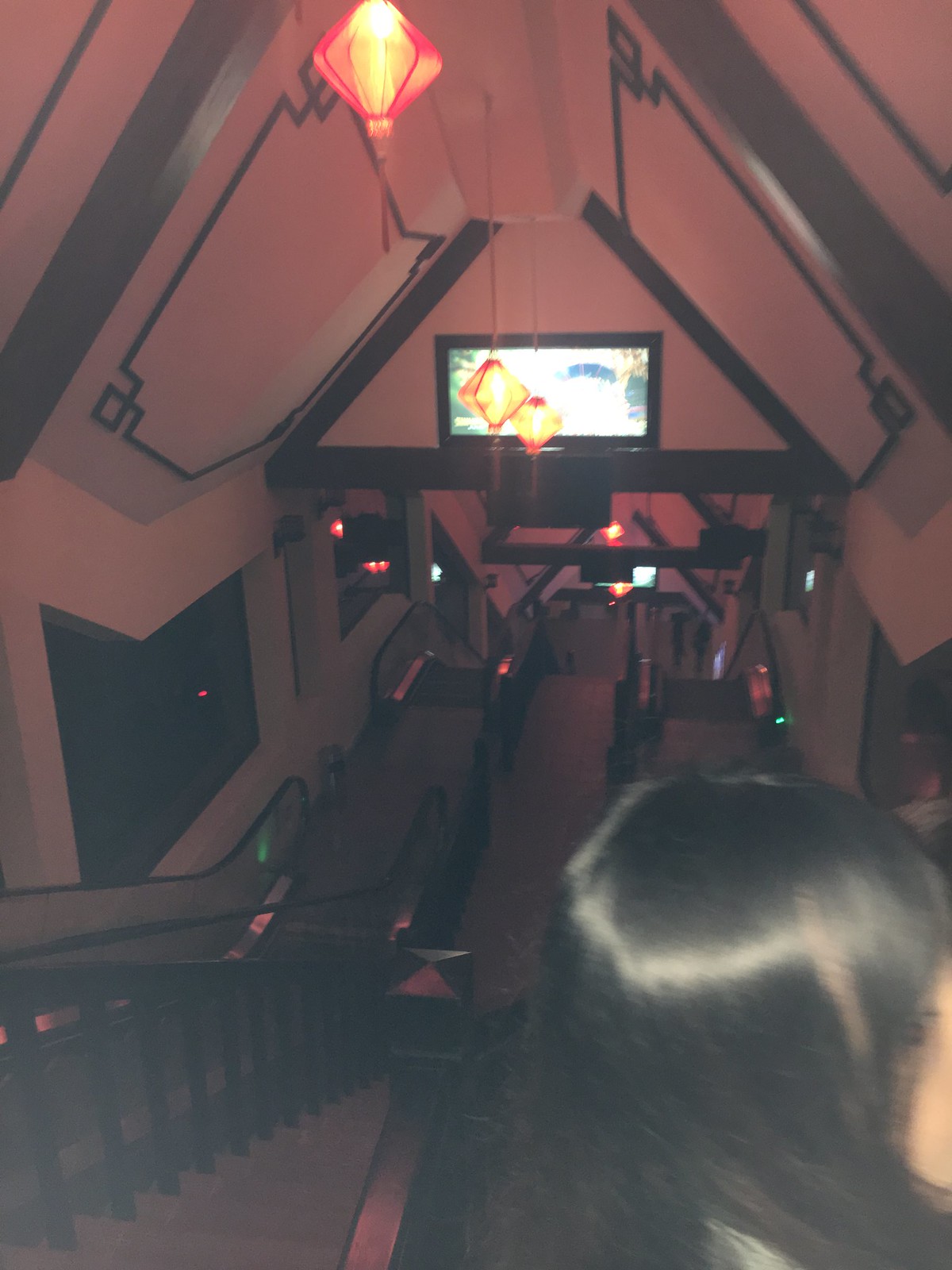This image portrays a dramatic view looking down into a multi-level, intricately designed stairwell bathed in a striking pink-tinged light. The vibrant hue, possibly emanating from the ceiling lights, casts an ethereal glow over the entire scene, accentuating the architectural details of the space. The ceiling itself is a cathedral-style design adorned with wood-like rafters forming triangular shapes as they descend, echoing the repeated triangular patterns of the steps below.

The stairs are made from a dark wood, nearly black, providing a stark contrast to the pink lighting. The stairwell spirals downwards with multiple landings, creating an illusion of endless descent. Suspended from the ceiling are unique lantern-style lights, with a yellow core surrounded by a red casing, and each light is finished with a tassel. These lights add an additional layer of visual interest and warmth to the overall composition.

To the left side of the image, windows punctuate the wall, but the true colors of the surroundings are obscured by the pink lighting. TV screens or monitors, outlined in black and lit up, are mounted at various levels, adding a modern touch to the classic architecture. The right side of the photograph includes an unintended element – the back of a person’s head with dark, shiny black hair partially obstructing the view. This human element provides a sense of scale to the grandiosity of the stairwell.

Overall, this image captures a captivating blend of classic architectural beauty and modern elements, rendered even more intriguing by the unusual pink lighting.